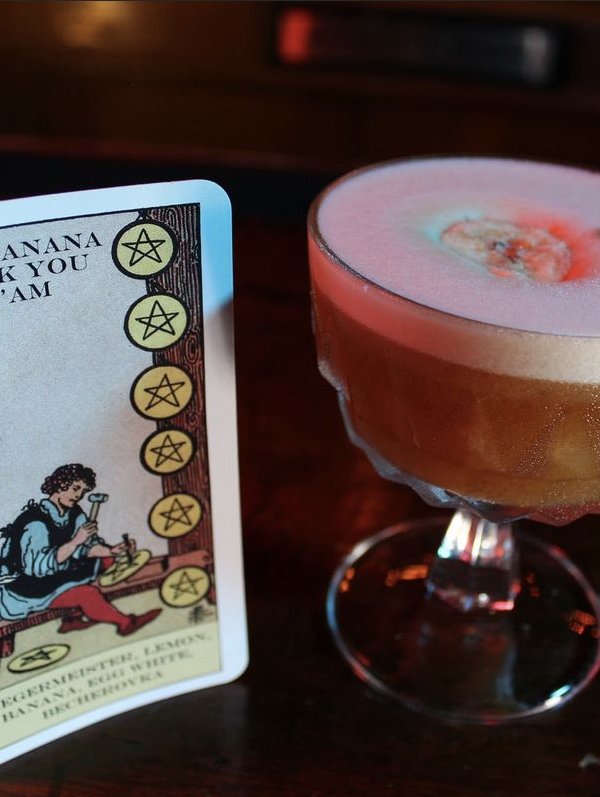This close-up photo captures two prominent objects resting on a dark brown tabletop. On the right side, there is a short-stemmed, large glass resembling a mini wine glass. It holds a multi-layered mixed drink with a light pink foam crowning the top. Below the foam, the liquid is a blend of colors, featuring a murky brown at the bottom and transitioning through variations of golden, white, and hints of orange and blue towards the top. Floating in the foam appears to be a small mass, possibly ice cream, with a pinkish hue on the right and white on the left.

To the left of the glass stands a tarot card in an upright position. The card's illustration depicts a man in medieval attire—a blue jersey with a black vest and pants, completed with red shoes—sitting on a bench and diligently chiseling a star into a circular object, likely a piece of wood or glass. The background of the card emphasizes a vertical brown tree trunk adorned with yellow star-filled circles. Black letters against a gray background mark the top and bottom of the card, with the bottom text being in a language other than English.